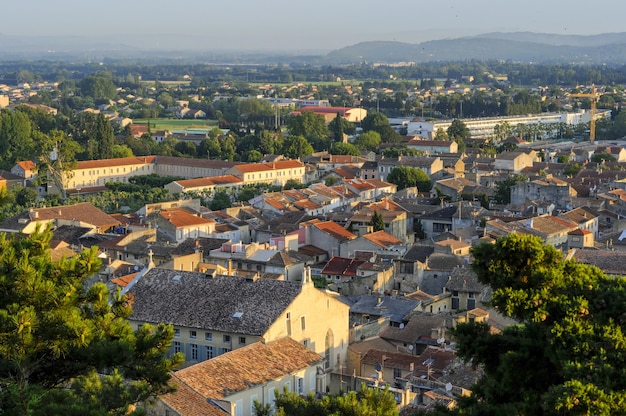This panoramic photograph captures a quaint town, likely situated in Europe or Mexico, viewed from a hillside. The scene is framed by evergreen trees in the foreground, adding depth to the composition. The town below is densely packed with buildings predominantly characterized by their red or orange-brown roofs, among various shades. These buildings are primarily constructed from light tan or golden-hued stone, evoking a historic charm.

In the mid-left portion of the image, a prominent U-shaped, two-story building stands out, possibly part of a school or campus, distinguished by its orange roof. Scattered throughout the town are patches of lush green foliage from different trees and bushes, providing a refreshing contrast to the earthy tones of the structures.

Towards the right in the distance, a long, modern white building is visible along with a yellow construction crane, hinting at ongoing development in the area. Further beyond, the landscape transitions into a vast, green field, with hilltops and a smoggy sky forming the backdrop. The combination of historical and contemporary architectural elements, along with the natural surroundings, lends a picturesque quality to the town nestled in this flat, expansive terrain.